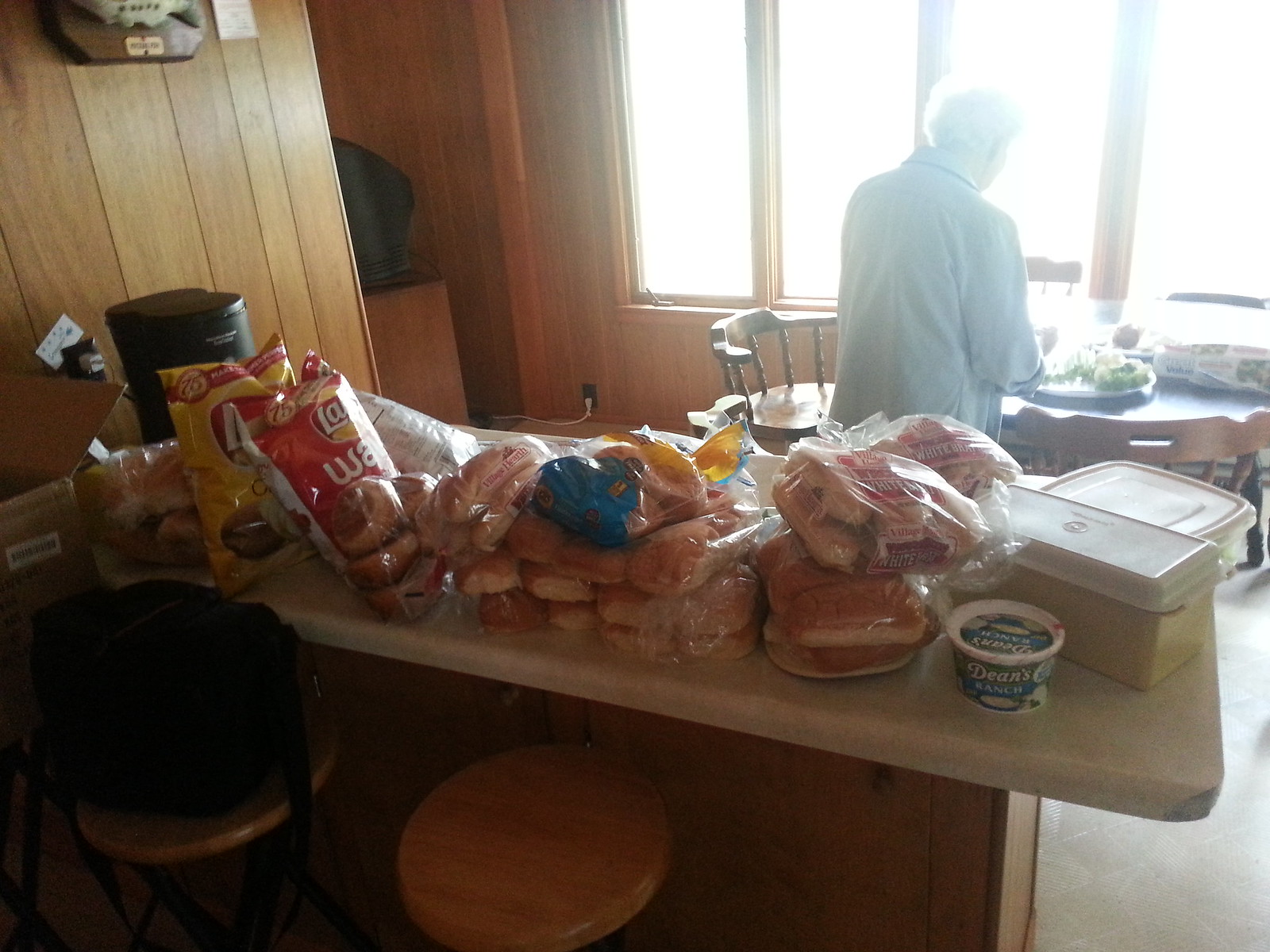This photograph captures the interior of an older individual's home, with a focal point on their kitchen area. At the forefront, there's a white, island-style countertop laden with groceries, suggesting the preparation for a picnic or a recent trip to the grocery store. The items on the counter include three packages of hot dog buns, several packs of hamburger buns, Lay's Classic potato chips in a yellow bag, Lay's Wavy potato chips in a red bag, and a container of Dean's ranch dip. To the front left, a black purse-like bag rests on one of the two wooden bar stools facing the counter.

In the background, the room is illuminated by sunlight streaming through several base-style windows. The walls are panelled with wood, adding a rustic charm to the space. An older person, distinguishable by their short white hair and dressed in a long-sleeved blue button-down shirt, stands with their back to the camera. They appear to be engaged with something on a small, old-fashioned wooden table and chair set situated near the windows. Scattered around them are various kitchen items, including rectangular and square plastic Tupperware containers. The overall atmosphere is homey and quaint, capturing a moment of domestic life.